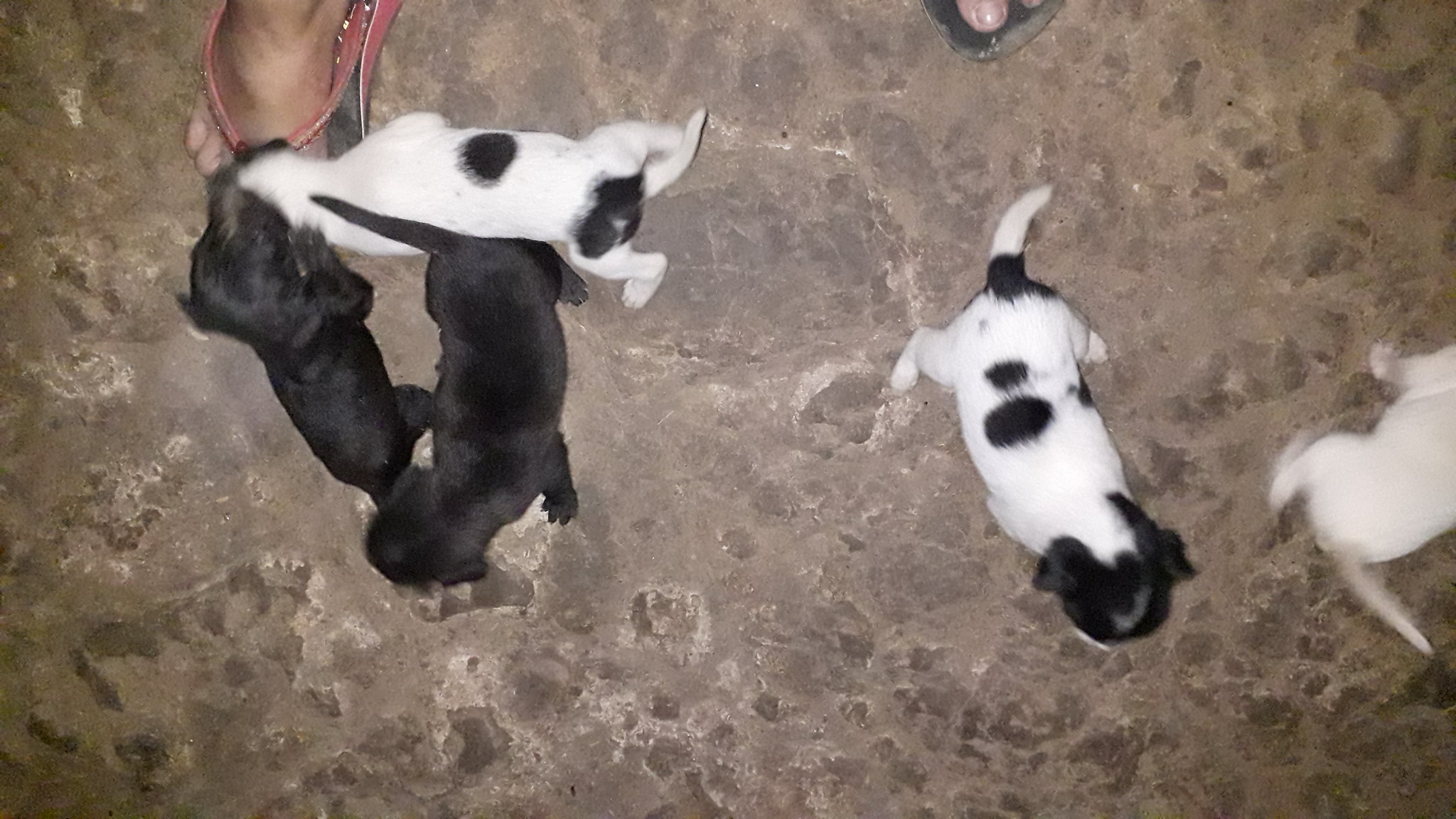The image captures a group of adorable puppies on what appears to be a beige-speckled, dirt-covered floor or rocky ground. There are six puppies in total, all seemingly from the same litter. The puppies include three white ones, two all-black ones, and one with a black-spotted white body and a black head. A pair of legs in pinkish, open-toed sandals adorned with rhinestones is visible in the background. The photo is taken from a wide angle, directly downward, providing a view of the puppies' bodies but not their faces, and it also shows another pair of feet in flip-flops, adding a sense of casual environment to the scene.